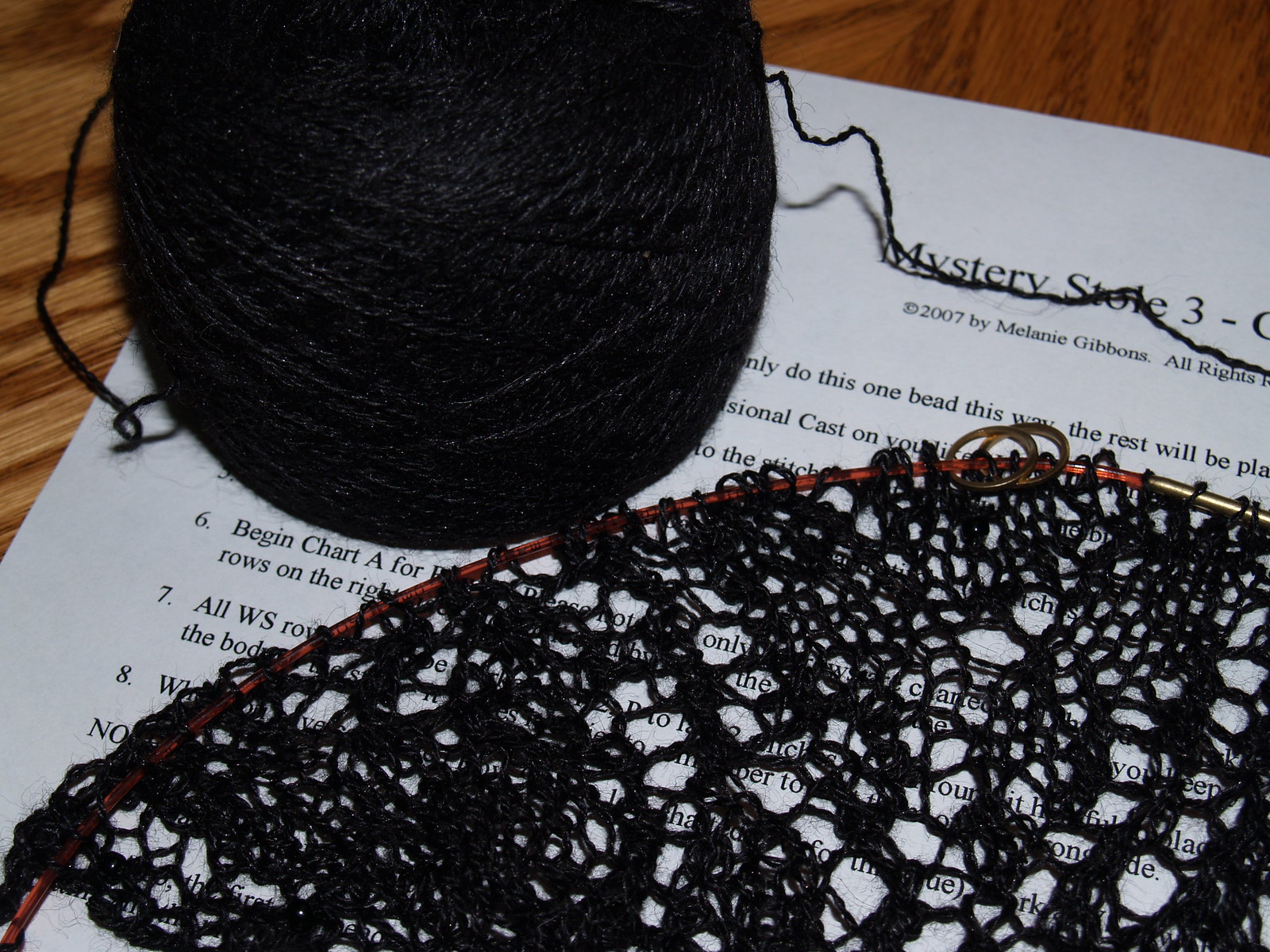The image showcases a detailed close-up of a crochet project in progress, laid out on a brown wooden table. Central to the scene is a white piece of paper, partially obscured by other objects, but legible enough to read "Mystery Stole Three, Copyright 2007 by Melanie Gibbons" at the top. The paper lists instructions numbered one through eight, though much of the text is hidden. Positioned at the upper left corner of the paper is a slightly unraveled spool of very thin black yarn. Adjacent to this is a copper-colored wire frame or hoop, intricately entwined with the same black yarn from the spool. This yarn has been meticulously crocheted into a delicate lace or doily-like fabric, forming an elegant pattern around the hoop. The contrast between the dark yarn and the bright copper hardware creates a striking visual on the simple backdrop of the table and instruction sheet.